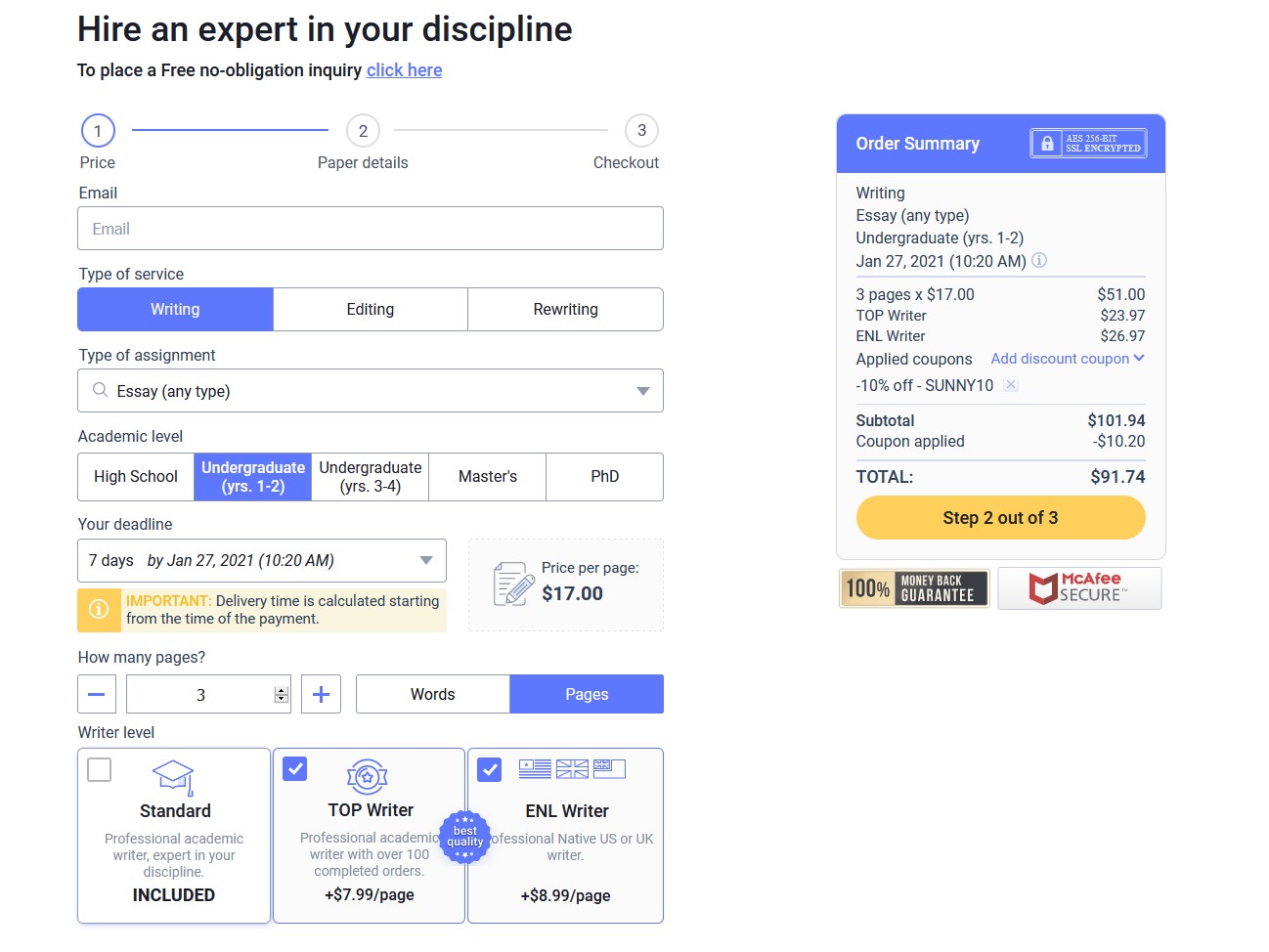In this image, the webpage prominently displays a call-to-action banner at the top offering users the option to hire an expert in their discipline. It invites visitors to place a free, no-obligation inquiry by clicking on a hyperlink labeled "Click Here," which opens in a new tab. To the right of the image, there are additional summaries and details pertaining to the services offered on this page. The breakdown of services includes charges for three pages at $17 each, totalling $51, with an additional "Top Writer" fee of $23.97. Applied coupons result in a 10% discount on the overall subtotal of $101.94, bringing the final total to $91.74 after the discount is applied.